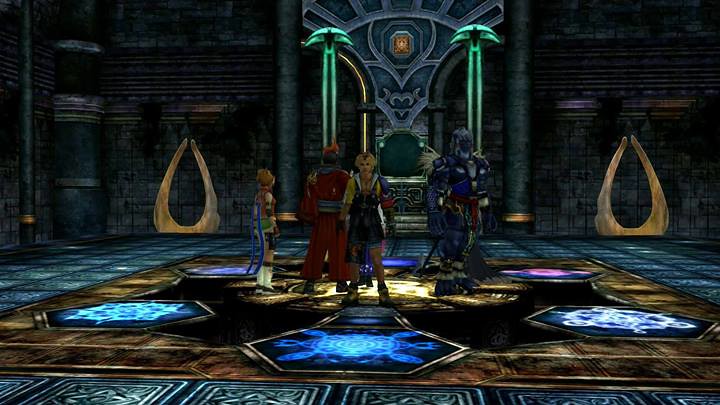This image depicts a screenshot from a fantasy RPG video game, reminiscent of the World of Warcraft era. The setting is a grand, intricately-designed space that suggests a castle or dungeon, characterized by detailed columns and likely marble construction. Central to the scene is a large, illuminated square panel on the floor featuring multiple geometric shapes and glowing sigils in various colors. There are four characters present, each distinctly attired, suggesting they come from different backgrounds or roles. Two characters stand on the left with their backs to the viewer, while the two on the right face forward. One of these characters, in the right-hand side, is notably a large, muscular blue figure with oversized hands. They stand on a section of the lit-up floor, which includes a prominent yellow circle highlighted within the square panel. Additionally, the room features green radiant lights and decorative elements that give it an altar-like atmosphere. Above this area, a throne is visible, adorned with a wolf-like gargoyle head crowned by a gem, enhancing the room’s majestic and mystical ambiance.